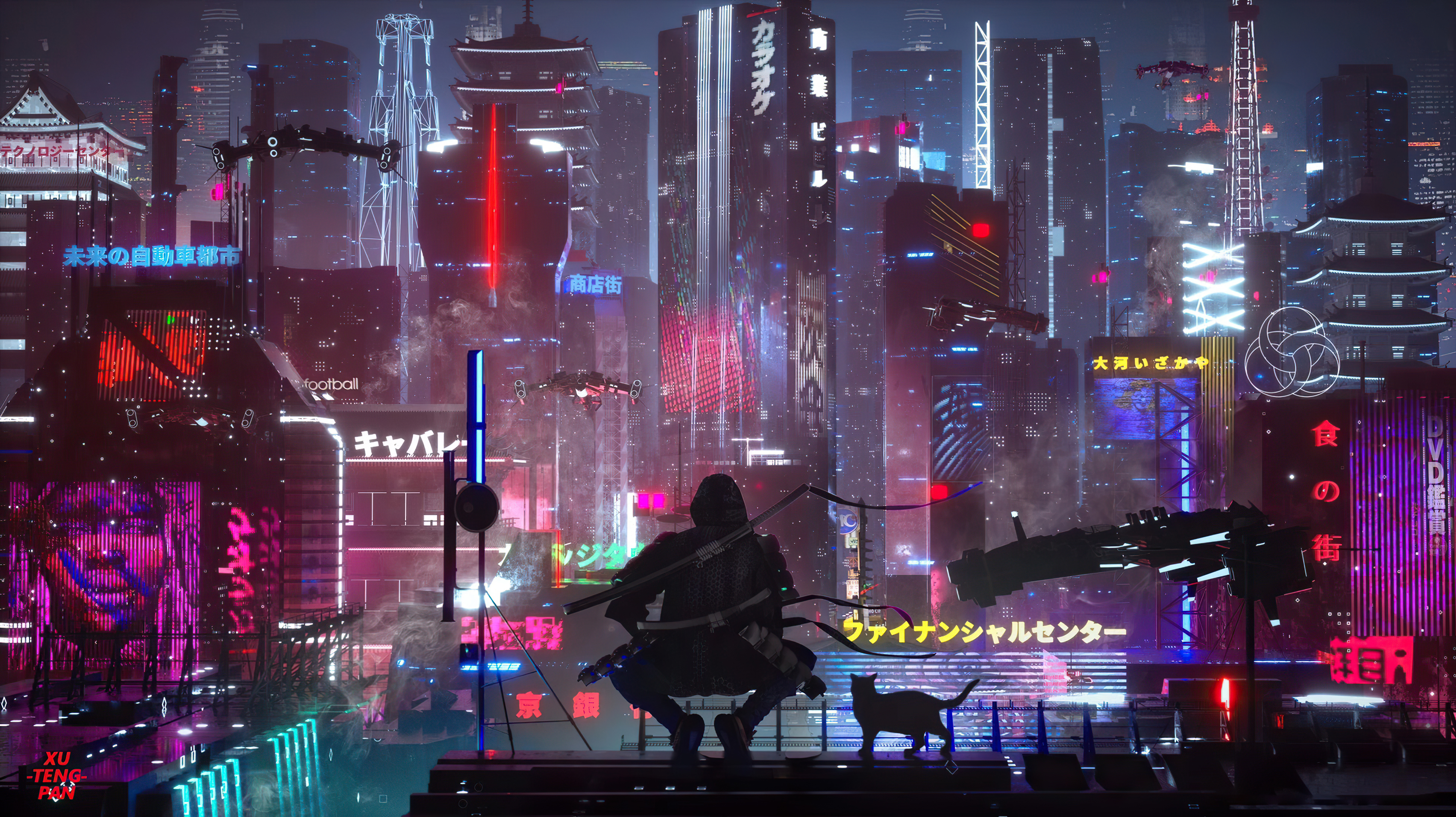A horizontally aligned, computer-generated image showcasing a futuristic Tokyo at night. The scene is bathed in vibrant, psychedelic hues of purples and blues, with numerous skyscrapers adorned with Japanese writing and dazzling lights. Among the illuminated cityscape, several flying ships or drones are noticeable in the night sky. Central to the image is a ninja dressed in black, seated on a bench with samurai swords crossed on their back. Beside the ninja, a cat sits attentively. On the lower left, there's a prominent screen displaying a pink, digital image of a woman, lending a cyberpunk feel to the setting. Additionally, the name "Xu Teng Pan" is printed in red letters in the lower left corner.